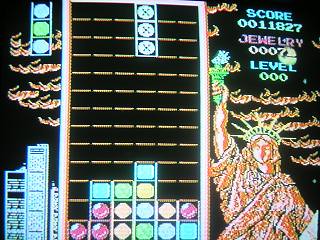This photograph captures a classic CRT television displaying a gameplay screen from "Magic Jewelry 2," a match-three puzzle game reminiscent of "Columns," running on the Nintendo Entertainment System (NES). The game appears to be a bootleg version, as suggested by the visual elements and overall aesthetic. On the screen, the iconic Statue of Liberty is visible, adding a unique flair to the game's interface. The scoreboard prominently shows the game's title, "Jewelry," and the current level, which is marked as level zero. Various colorful puzzle pieces are scattered at the bottom of the game field, with the player actively clearing substantial sections of them. This image encapsulates a nostalgic moment in retro gaming, highlighting both the game’s mechanics and the experience of playing on vintage hardware.